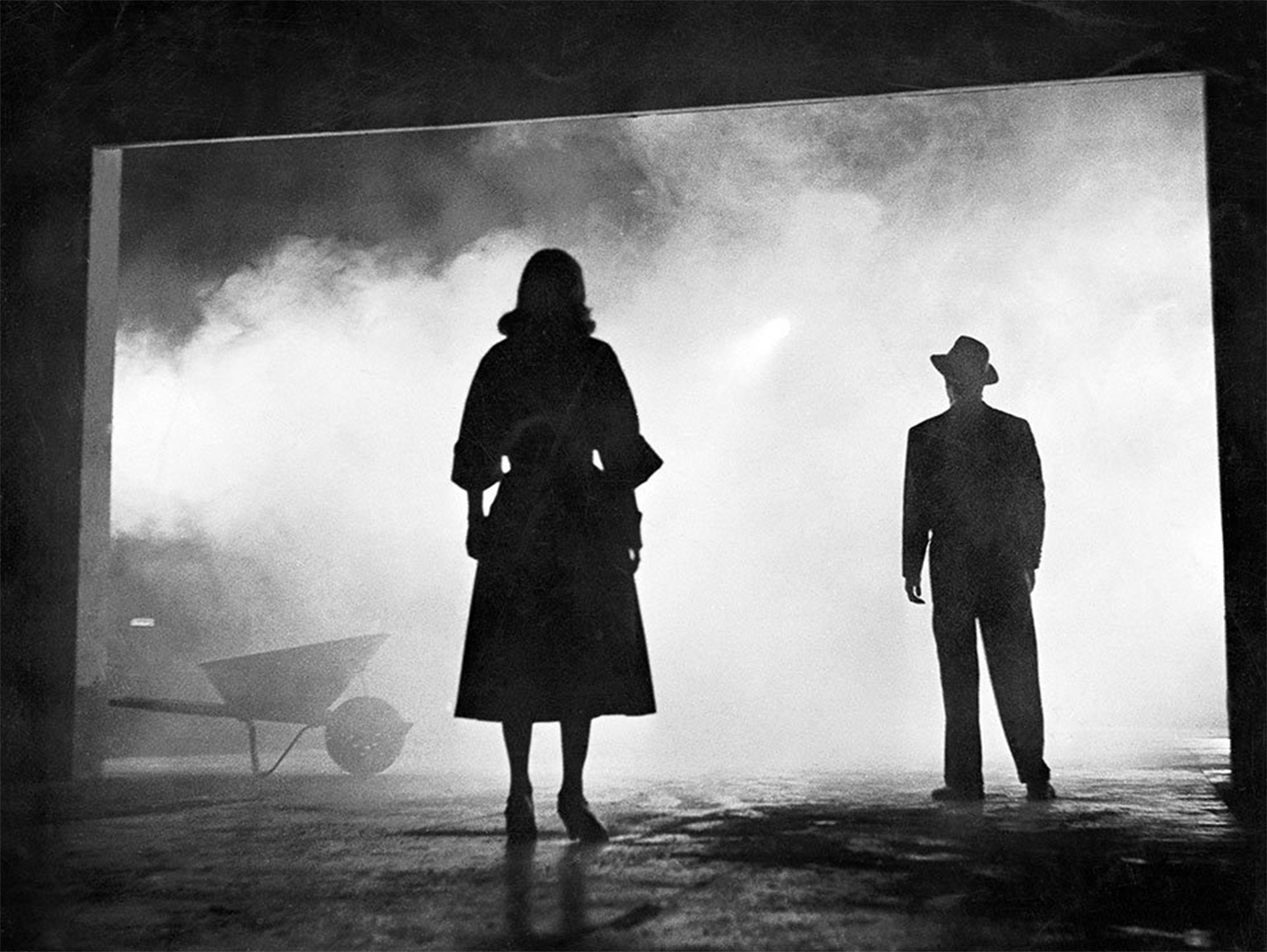This detailed black-and-white photograph, likely a still frame from an old film reminiscent of classics like Casablanca, captures a striking scene where two silhouetted figures stand at the threshold of a large garage-like opening. The scene is enveloped in a mysterious white fog that brightens the background, contrasting sharply with the dark foreground and the silhouettes. On the right, a man in a hat and suit gazes upward into the fog, while on the left, a woman in a long-sleeved, puffy dress and high heels looks in the same direction. The garage floor at the bottom is visible, appearing dark and dotted with wet, reflective spots. At the left edge of the opening, a wheelbarrow adds to the atmospheric, somewhat eerie setting of the image.